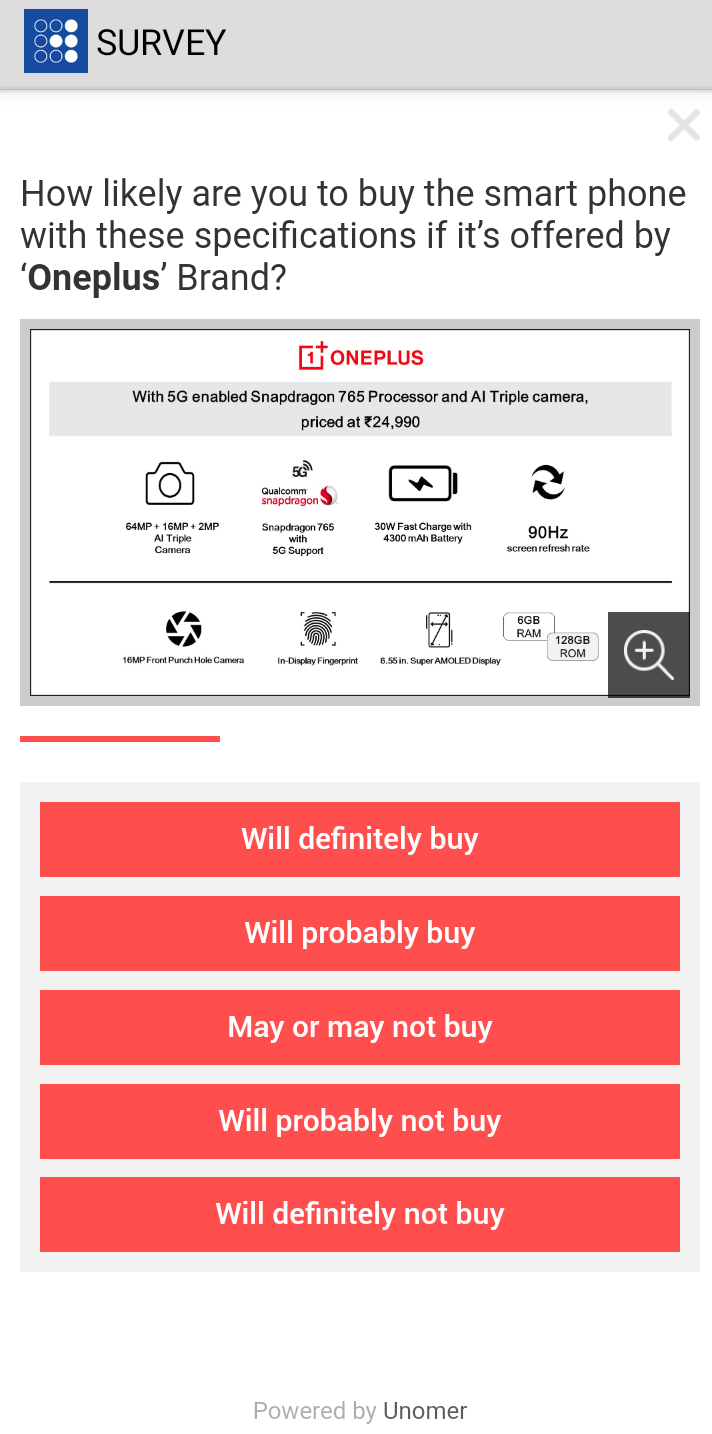The image is a survey related to a OnePlus smartphone, prominently featuring a blue background with a grid of nine dots, with some dots colored white and one in the middle of the last row highlighted. The survey poses the question: "How likely are you to buy a smartphone with these specifications if it’s offered by the OnePlus brand?" The specifications of the phone in question include:

- 5G enabled Qualcomm Snapdragon 765 processor
- AI triple camera system: 64MP + 16MP + 2MP
- 30W fast charging with a 4,300 mAh battery
- 90 Hz screen refresh rate
- 16MP front punch-hole camera
- In-display fingerprint scanner
- 6.55-inch Super AMOLED display
- 6GB RAM and 128GB internal storage
- Priced at ₹24,990

The survey provides five response options in red blocks: "Will definitely buy," "Will probably buy," "May or may not buy," "Will probably not buy," and "Will definitely not buy." At the bottom of the image, it is marked as "Powered by Unomer."